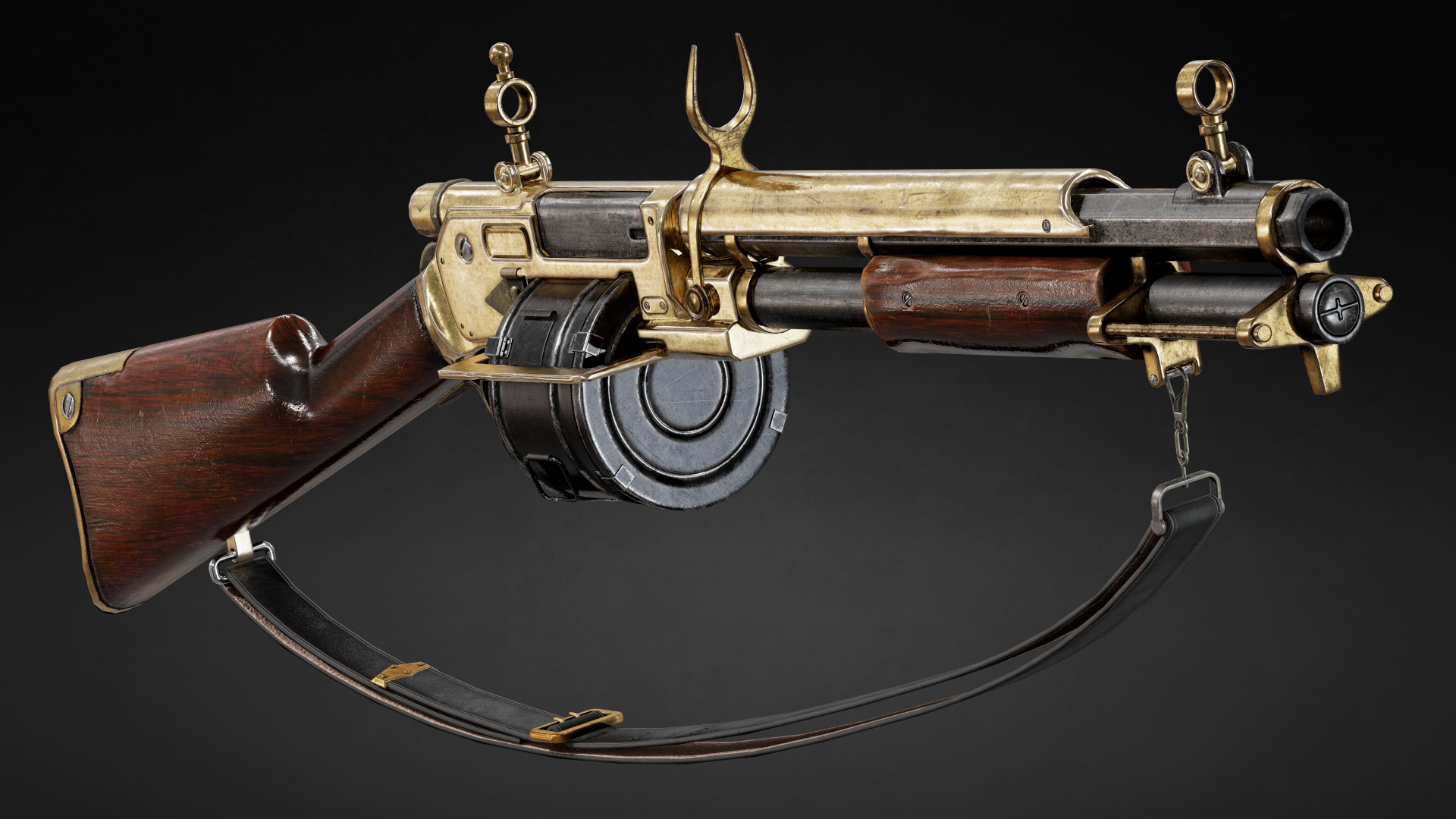This photograph captures a meticulously preserved antique gun, possibly transitional between a musket and a machine gun. It showcases a beautifully finished wooden stock with brass accents, including a brass plate at the back and additional brass plating extending underneath the top of the stock. The gun features a unique round rotary magazine and an elaborate brass sighting system. The barrel, which appears octagonal and darkly patinated or black, is partially encased in brass that covers about two-thirds of its length. It incorporates a pump-action mechanism with a wooden handle, allowing shells to be loaded and chambered manually. Additional details include a brass shroud around the barrel, brass brackets securing the tube for the mechanism, and a distinctive horseshoe-type brass sight. The entire assembly is adorned with brass and gold elements, and includes a leather strap with brown accents. The photograph is set against a dark gray background that emphasizes the gun’s intricate design and historical significance.